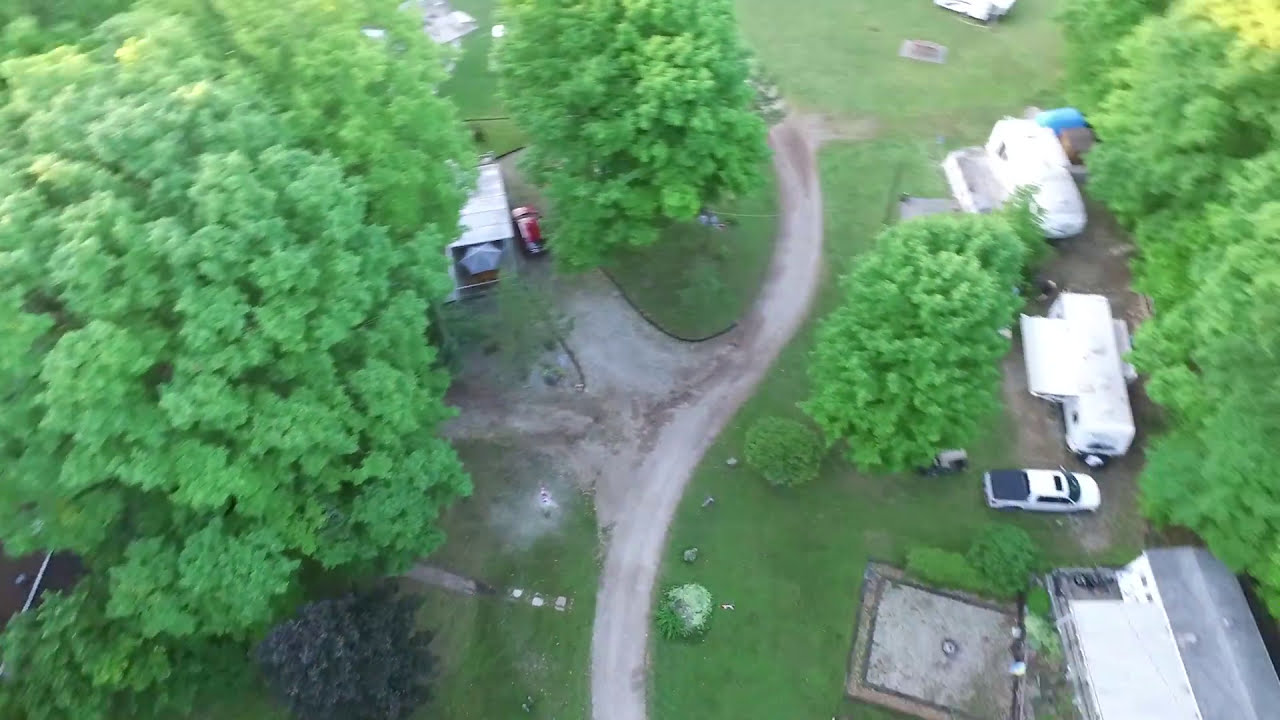This aerial photograph captures a slightly blurry, rural trailer park area during the daytime, providing a wide view of the landscape and its features. The image prominently displays a network of dirt and lightly paved roads running through the scene, with one main road entering from the bottom center and forking in different directions: straight ahead into dense tree cover, sharply to the left, and on a curved path also to the left. 

Amidst scattered, tall trees, which appear throughout the image and obscure some details, distinct elements include a concrete pad nestled between the trees on the right and several mobile home structures. On the right side of the photograph, there are three white campers aligned, with one featuring an awning extended. Between the first and second camper, a white truck is visibly parked. The second camper appears less permanent, suggesting it could be moved. Toward the upper left third and under tree cover, there seems to be a box truck near a red vehicle parked on another dirt road. 

The area has a somewhat rundown appearance, indicative of a low-income, rural setting. Despite the blurriness and slight motion blur, likely from being taken by a drone or a fast-moving aerial device, the photograph effectively conveys the layout and character of this trailer park community surrounded by extensive greenery.